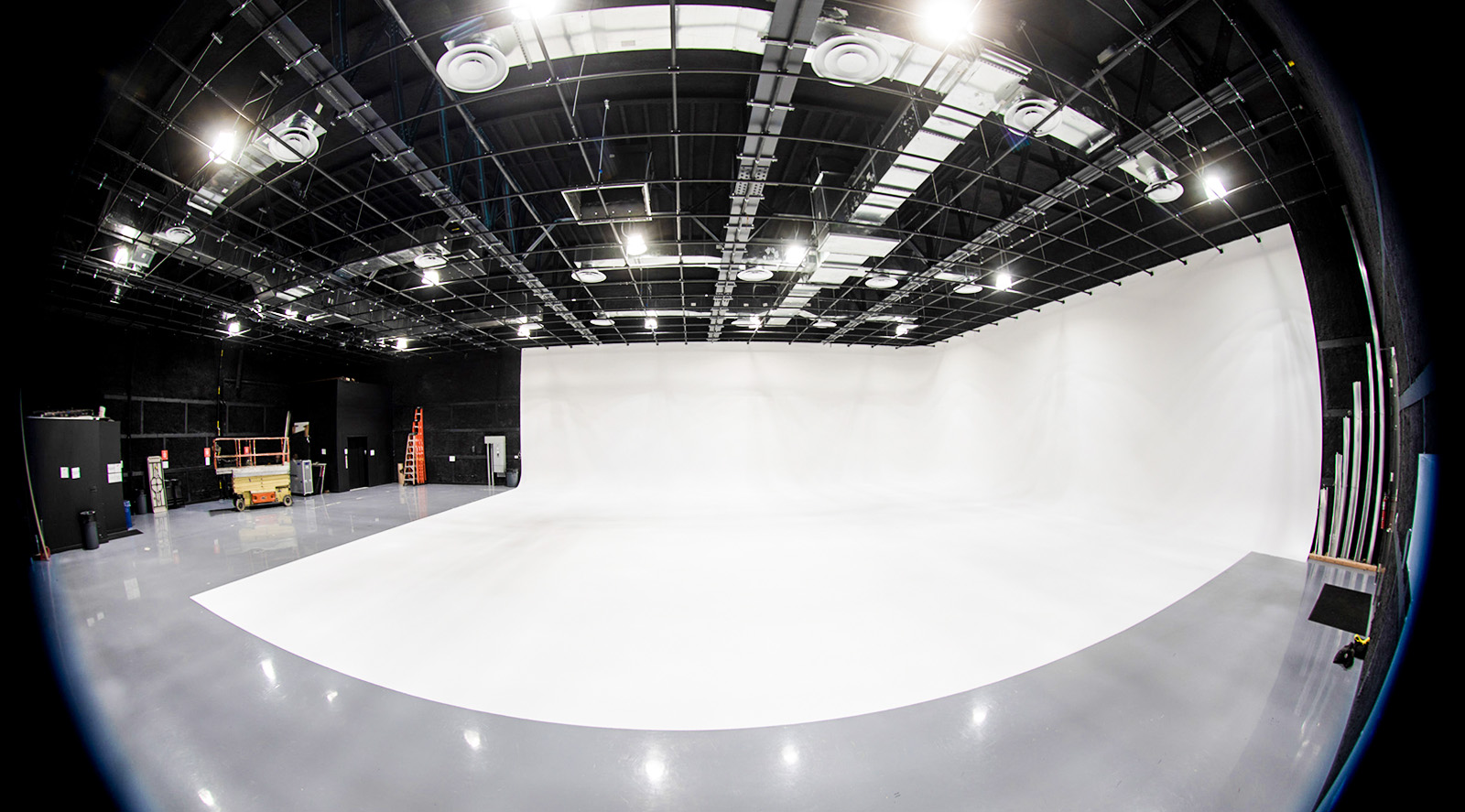This image, captured through a fisheye lens, shows a concave view that balloons outwards towards the center. The scene is set against a black background which, along with the lens distortion, gives the entire frame a rounded appearance. The setting appears to be an indoor space that could be an ice arena, warehouse, or possibly a stage production area. The floor looks like an ice surface or a shale gray floor, illuminated by bright overhead lights affixed to a steel girder ceiling structure. Scattered around are various pieces of equipment including an orange and yellow forklift cart on the left side, and white ladders visible in the background. The overall color scheme of the image is predominantly black and white, with occasional silvers and white lighting reflections off the ground. There is a large white backdrop, vents at the top, and other assorted backstage-looking elements, heightening the cold and sparse atmosphere of the scene.